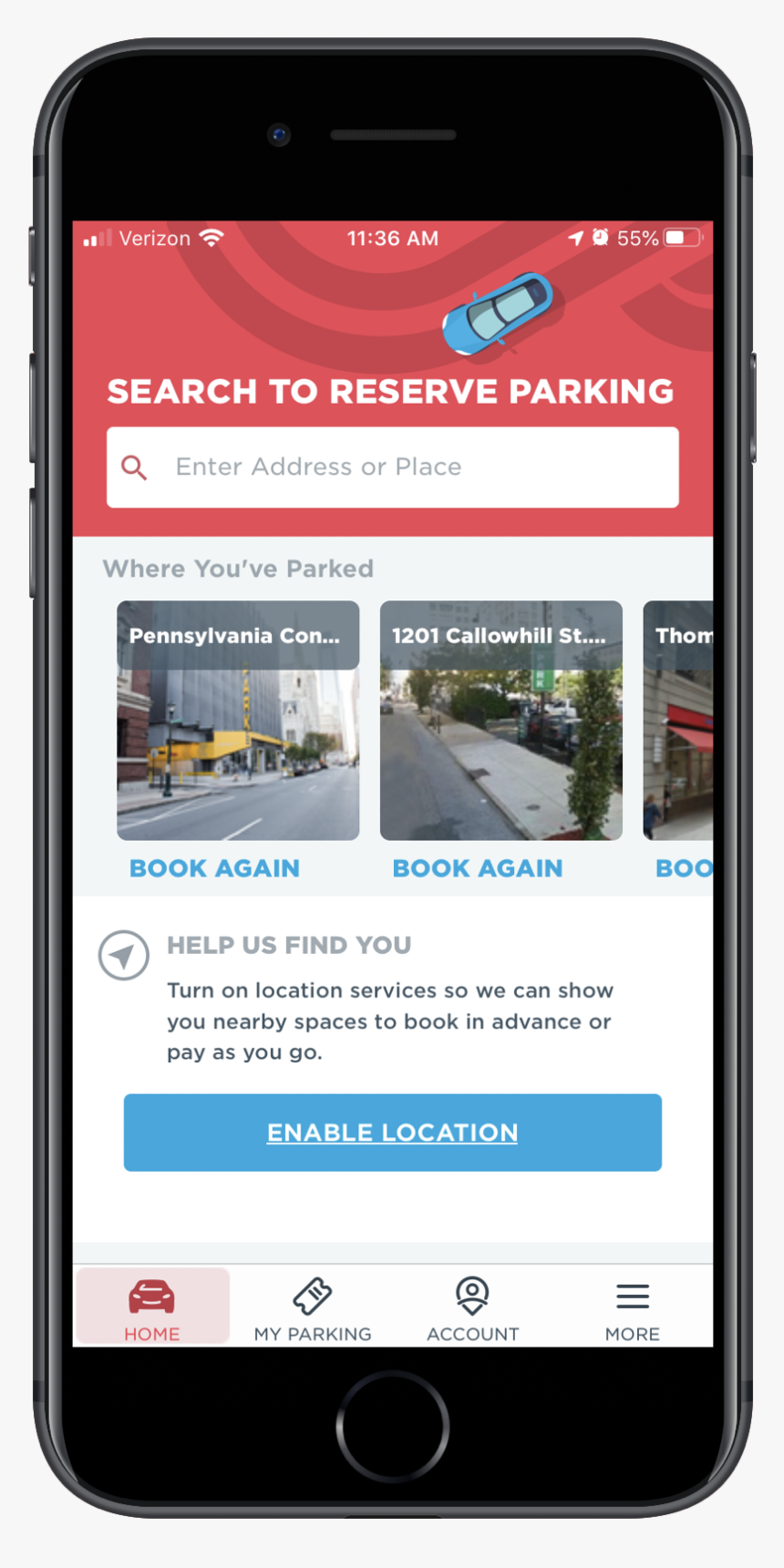A mobile phone screen displaying a parking app is shown in portrait format. The image includes visible elements of the phone itself: black strips at the top and bottom with the home button encased in a protective cover. The right side of the case features a solitary button, while the left side has three buttons, the uppermost one being slightly smaller.

At the screen's top, the status bar reveals: two filled signal bars out of four, the Verizon carrier name, a fan-shaped signal strength icon, and the device time—11:36 a.m. Further to the right, there are four symbols within a red banner: a northeast-pointing arrow, an alarm clock, the text "55%" indicating the battery level, and a battery icon slightly over half full. The red banner also showcases curved gray lines resembling roads, with a blue cartoon saloon car featuring a panoramic roof positioned on one of these lines. The banner's text reads, "Search to reserve parking," accompanied by a search bar prompt, "Enter address or place."

The remainder of the app screen has a white background. To the left, in gray text, the section labeled "Where you've parked" presents three previously visited locations displayed as photos. The first photo shows a street scene with a tall building and the partially visible text "Pennsylvania C.O.N." indicating it is likely in Pennsylvania. The second image, captioned "1201 Callow Hill S.T.," depicts another street scene. The third photo, slightly obscured, shows a store with an awning and the partial name "T.O.M." Beneath each photo is a blue "Book again" button. 

Further down, instructional text reads, "Help us find you. Turn on location services so we can show you nearby spaces to book in advance or pay as you go." This is accompanied by a filled-in arrow icon in a circle next to the word "Help." Below this, a blue "Enable location" button with white text and underline is prominently displayed.

At the bottom of the app interface, there are four icons from left to right—Home, My Parking, Account, and More. Each icon has accompanying illustrations: a red front-facing car (Home), a parking ticket (My Parking), a person inside a teardrop shape (Account), and three vertical lines (More).